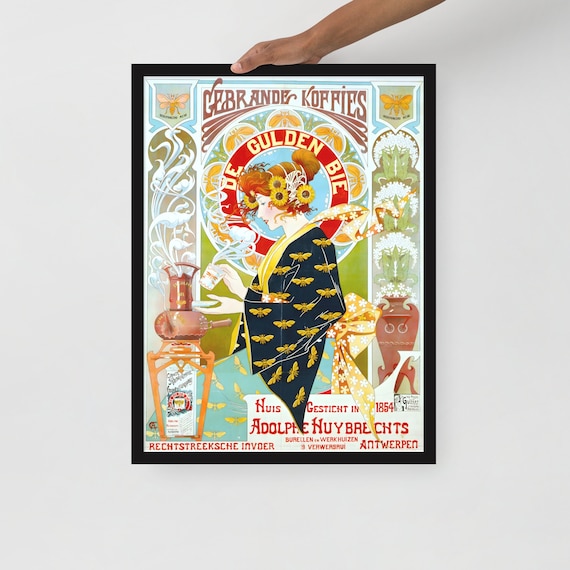The image displays a vibrant, framed artwork held by a hand visible from the top, appearing against a digital backdrop, similar to an Amazon listing display. The black-framed piece showcases a rich, multicolored design with prominent elements and foreign text, "Gebrande Coffees," at the top. Central to the artwork is a woman's head with flowing red hair adorned with a variety of flowers, encased within a red circular pattern. She is attired in a blue robe decorated with yellow or gold bees. The artwork features green floral patterns and additional text "DE GULDENBIE" towards the middle and "Adolph Hoibrex" in red at the bottom, along with other hard-to-recognize lettering. This detailed piece could be promotional material for a shop or an event somewhere in Europe, possibly Antwerp.